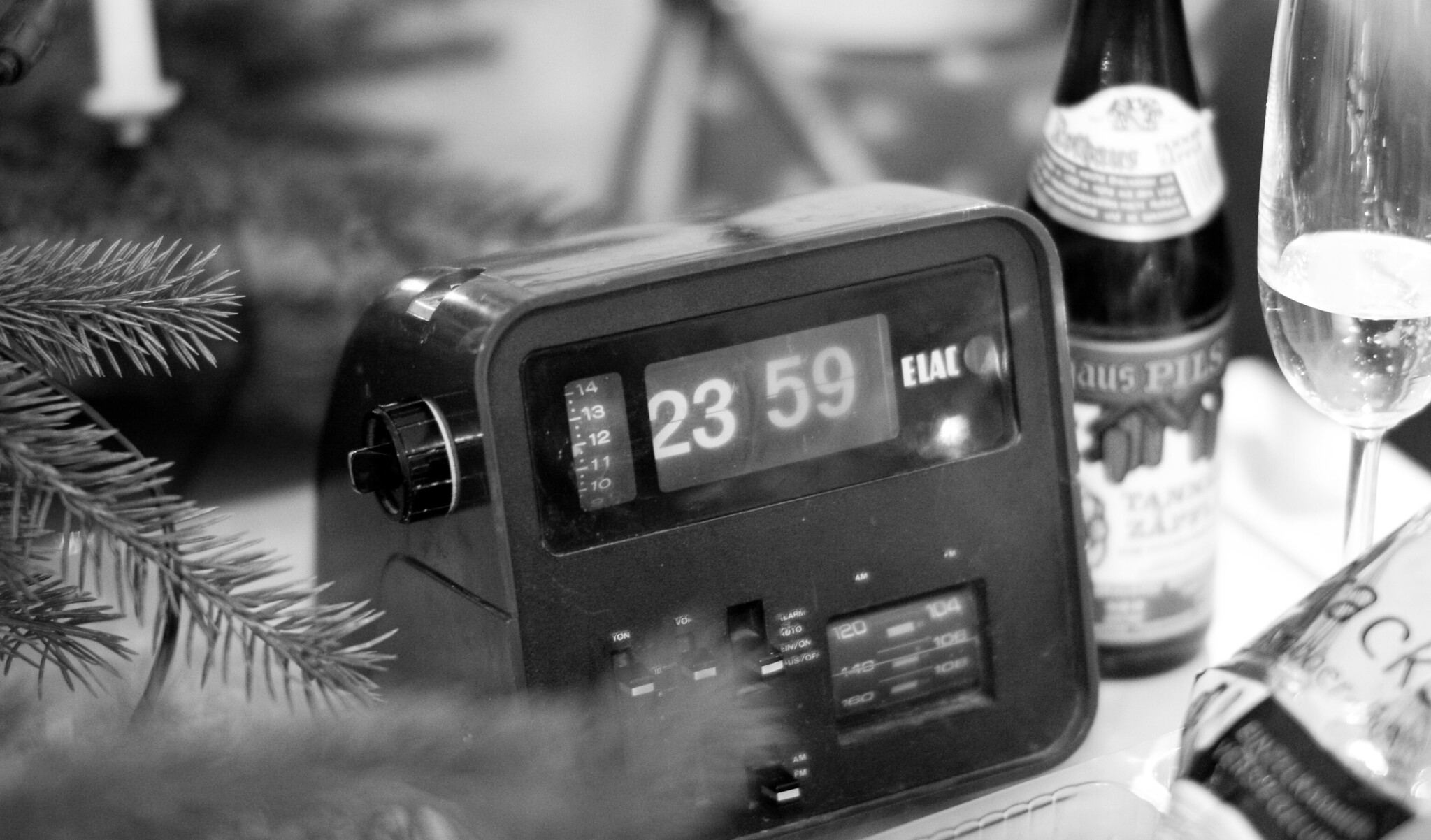This image is a detailed black-and-white photograph depicting a still life scene on a table. In the center, there is a vintage analog alarm clock with a square design and black detailing, displaying the time 23:59 in military time. The clock features several dials and buttons: a prominent dial on the left ranging from 10 to 14, another set of numbers from 100 to 120 at the bottom, and the white letters "ELAC" on the right side. To the left of the clock, a slightly blurred pine tree is partially visible, with pine needles encroaching into the frame. On the right side of the table sits a bottle of craft beer labeled "PILS" and a partially filled champagne flute. The background is out of focus but hints at a tranquil, perhaps forested, setting enhanced by the soft blur of a tree in the back left. A bag of food can also be discerned in the lower right corner.